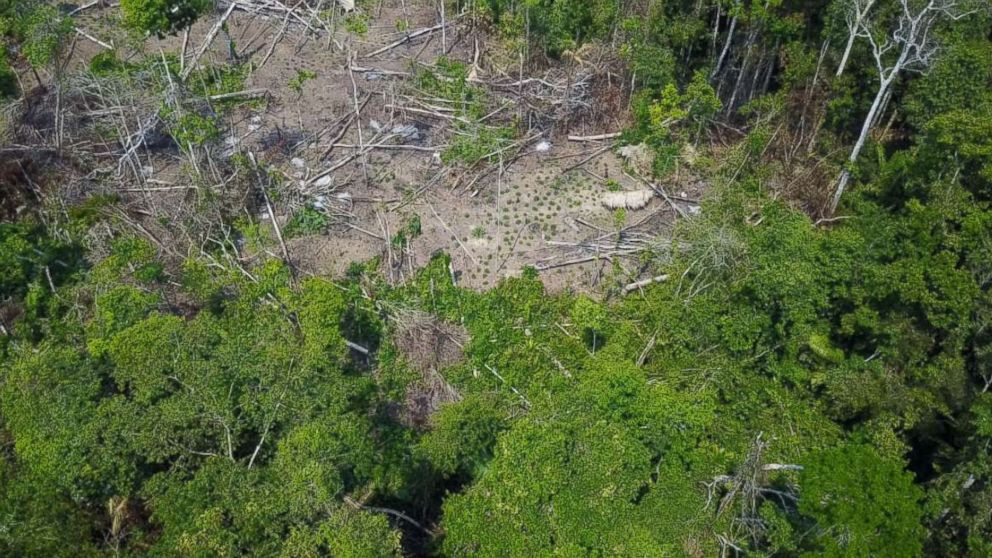The image presents an aerial view, possibly taken from a drone or helicopter, capturing a large circular clearing in the middle of a dense forest. The ground in the clearing is a mixture of brown dirt and sandy texture, interspersed with small shrubs and patches of green grass. Fallen trees, characterized by their gray, whitish trunks, and logs without branches or leaves, are scattered haphazardly across the clearing, indicating a logging operation. Around the clearing, the verdant, mature forest is visible, with tall trees and lush green canopies forming a dark green upside-down arch from the bottom of the image. A few gray stones dot the ground in the clearing, and there might be glimpses of simple structures or straw. The overall contrast between the open, desolate center and the vibrant, thriving forest around it is stark and evocative.